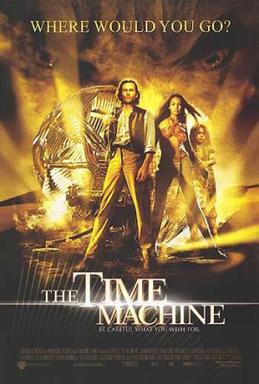This captivating poster, designed to advertise a movie or a book, features an ominous backdrop dominated by a monstrous creature's face. The creature’s eyes, rendered in a haunting yellow-brown hue, are intensely focused downward, as if scrutinizing the scene below. At the center of the composition, a luminous sphere radiates light, illuminating three central figures: a man, a woman, and a child. They stand with their legs arranged to form an 'A' shape between them, suggesting unity and strength. At the bottom of the poster, the title "THE TIME MACHINE" is prominently displayed in white capital letters, with "TIME" in a larger font, followed by the slightly smaller "MACHINE," and the smallest "THE" preceding them both. The top of the poster poses an intriguing question in bold capital letters: "WHERE WOULD YOU GO?" This thought-provoking query invites viewers to imagine the endless possibilities within the depicted time-travel adventure.